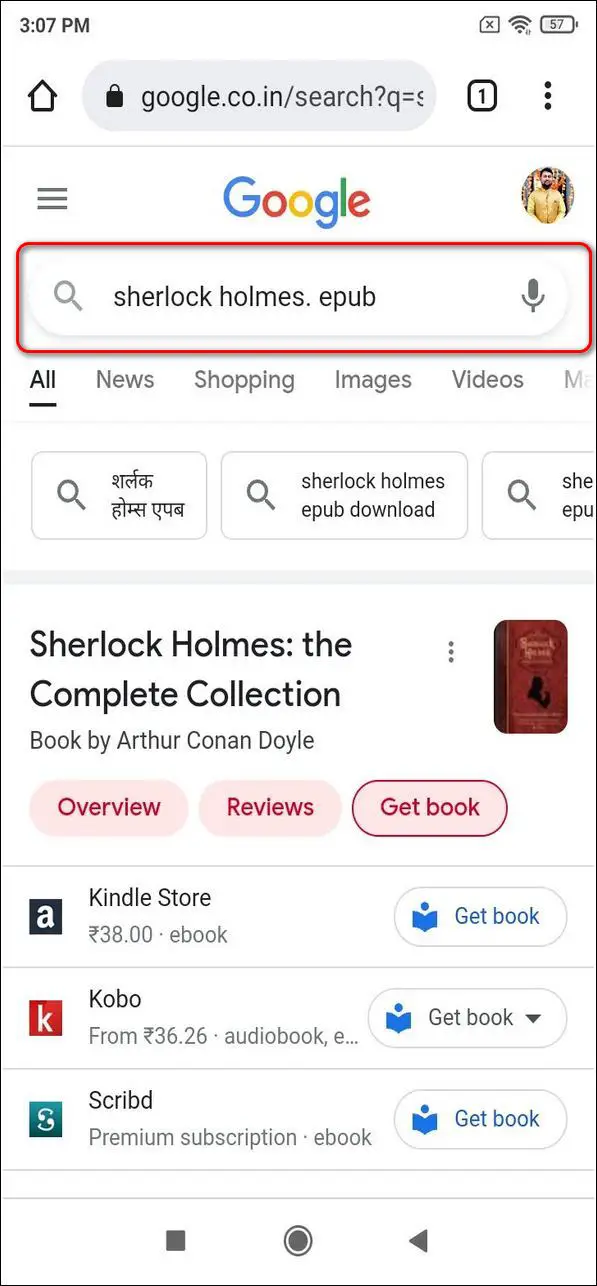This screenshot from an Android phone displays the Google Chrome app. At the top left corner, the current time is shown as 3:07 p.m., and to the right of the time, the Wi-Fi signal strength and battery level (at 57%) are displayed. Below the time indicator, there is the Chrome home button and a partially visible URL: "google.co.in/search?q=".

The primary browser tab shows three vertical dots signifying the settings menu. Enclosed in a red rectangular highlight is the search input field with the text "sherlockholmes.epub" next to the magnifying glass icon. Adjacent to the search field is a microphone icon. 

Below the search bar, the 'All' tab is underlined, with other tabs labeled 'News', 'Shopping', 'Images', and 'Video' appearing next to it. 

The top search result displayed is titled "Sherlock Holmes: The Complete Collection" by Arthur Conan Doyle. This result includes an oblong, pink highlight with buttons labeled "Overview," "Reviews," and "GetBook" (the latter is highlighted).

Beneath this, the Kindle Store offers the e-book for 38 Indian Rupees, with a 'GetBook' button beside it. Below the Kindle Store option, the Kobo option is listed, offering an audiobook for 36.26 Indian Rupees, also displaying a 'GetBook' button. The entry for 'Scribd' follows, indicating it as a premium subscription for e-books and featuring yet another 'GetBook' button.

At the bottom of the screen, there are controls for voice recording, with a record button, stop button, and rewind button.

Overall, the screenshot captures an in-depth view of a search query for "sherlockholmes.epub" on the Google Chrome app on an Android device.